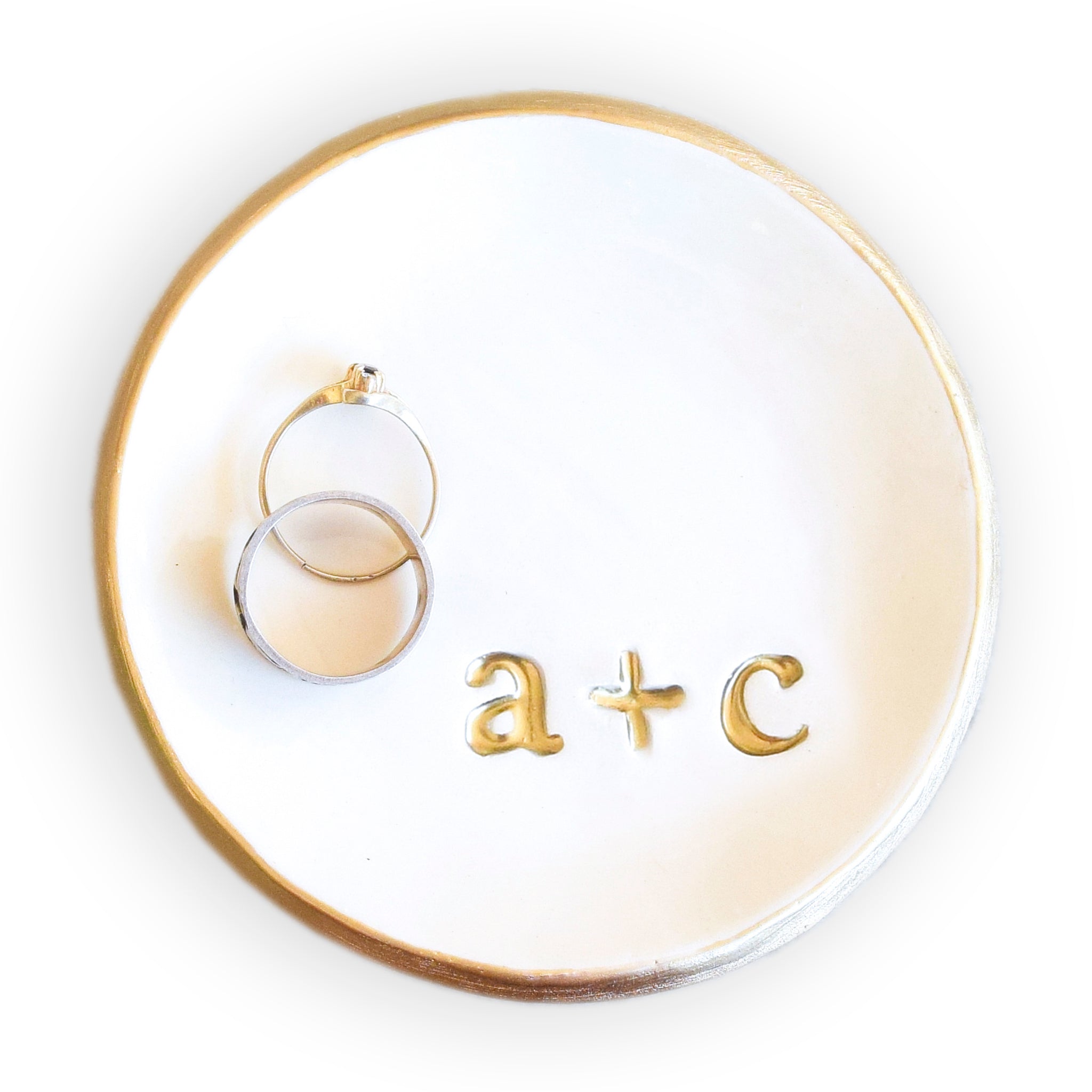The image depicts a round, white ceramic dish with ornate gold trim on its edges. The golden trim transitions from gold to brown as it encircles the dish, adding a touch of intricate detail. Inside the dish, towards the right, are gold inscriptions reading "a + c," likely indicating the initials of two individuals. To the left of the inscriptions are two rings: a sleek silver band, presumably a man's wedding band, resting on top of a more elaborate gold ring, likely a woman's wedding ring. The gold ring appears to have a gem, though the exact details are obscured by the angle. The dish sits against a white background, possibly indicating a product catalog image, with light reflecting off the gold trim, adding a gleaming effect.